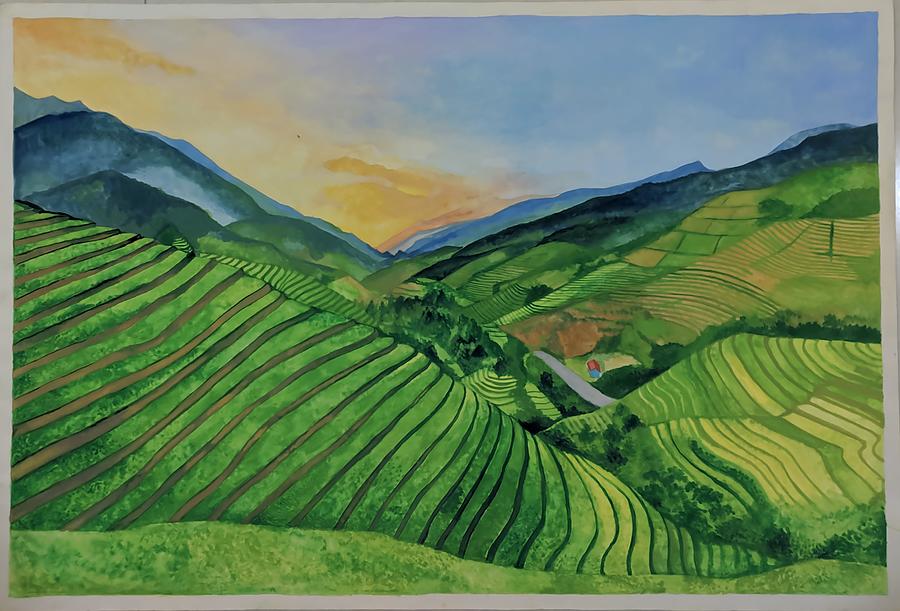This rectangular watercolor painting, measuring approximately five to six inches wide by four inches high, captures an exquisite landscape scene. Framed by a light gray border with a faint shine, possibly from a metal edge, the artwork prominently features a verdant valley nestled between terraced hills. These terraces, marked with alternating brown steps and green tops, suggest fields possibly used for rice or grape cultivation. At the center-bottom of the painting, a small gray pathway winds its way through the landscape, leading to a tiny blue and red figure that might represent a barn or house.

In the background, the scenery transitions into blue mountains, and the sky above exhibits a gradient from a yellow hue on the left, suggesting a sunset, to a blue expanse on the right, interspersed with sporadic clouds. The overall palette of the painting ranges from the dark green tops of the hills to the lighter greenish-blue shades at their bases, creating a rich tapestry of color that enhances the depth and beauty of this serene rural vista.